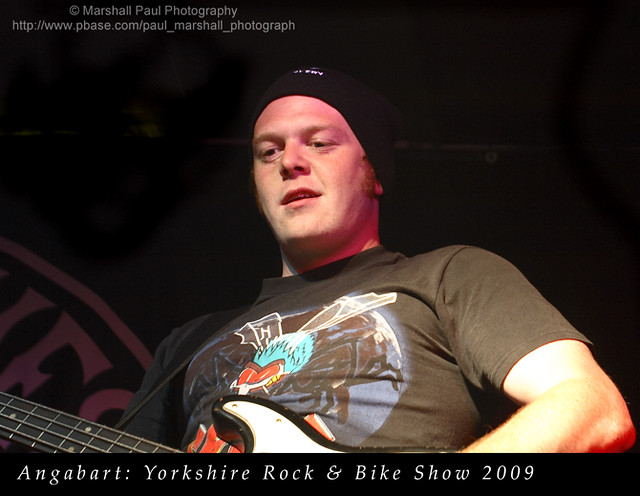This photograph captures a white man playing a bass guitar at the Yorkshire Rock and Bike Show 2009. He is seen standing on stage, the black background behind him adorned with a large white logo. The image features a copyright notice in the upper left corner reading "Marshall Paul Photography" with the website "http://www.pbase.com/paul_marshall_photograph." The man is wearing a black beanie with white lettering and a black t-shirt emblazoned with a cartoon fly or bug, which has blue wings and red eyes. His face is clean-shaven with brown hair and eyes, focused intently on his guitar playing. Visible from the chest up, the guitar’s neck and part of its body, which is black with a white overlay, can be distinctly seen. At the bottom of the photograph, in white text, it reads "Angabart, Yorkshire Rock and Bike Show 2009."